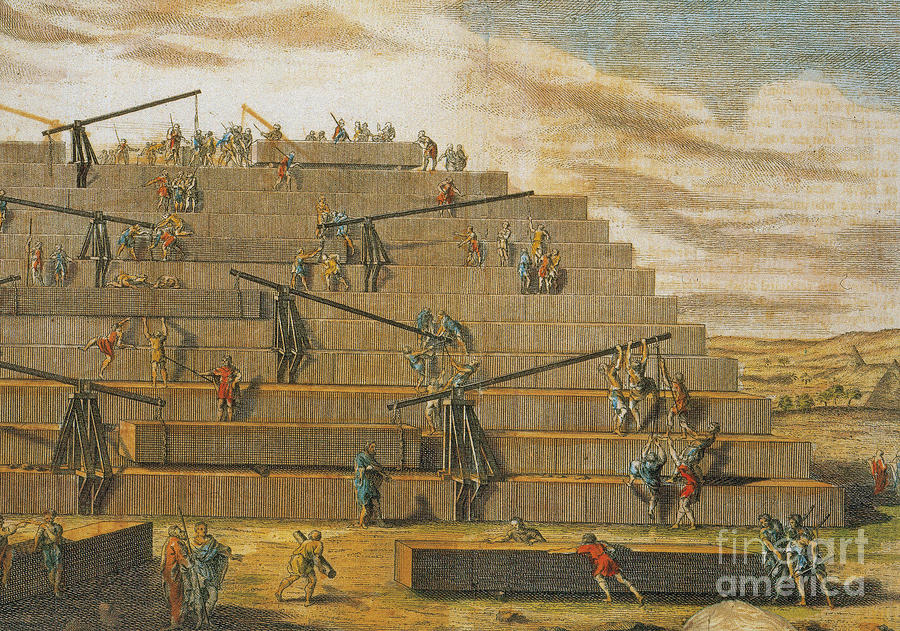This image is a detailed, color illustration in landscape style, produced by Fine Art America, identifiable by the logo in white on the bottom right corner. It depicts an ancient construction site, presumably in Egypt or Sudan, where dozens of workers clad in robes of varying colors—red, blue, and yellow—are collaboratively constructing a giant pyramid. The structure has visible stepped layers, suggesting that construction is about halfway complete. These laborers use cranes, pulleys, and levers to lift and position large stone blocks onto the pyramid, demonstrating a sophisticated and labor-intensive process. The pyramid occupies the majority of the image, reaching about three-quarters up, with partly cloudy skies filling the remaining upper portion, creating a vivid and historically rich scene.